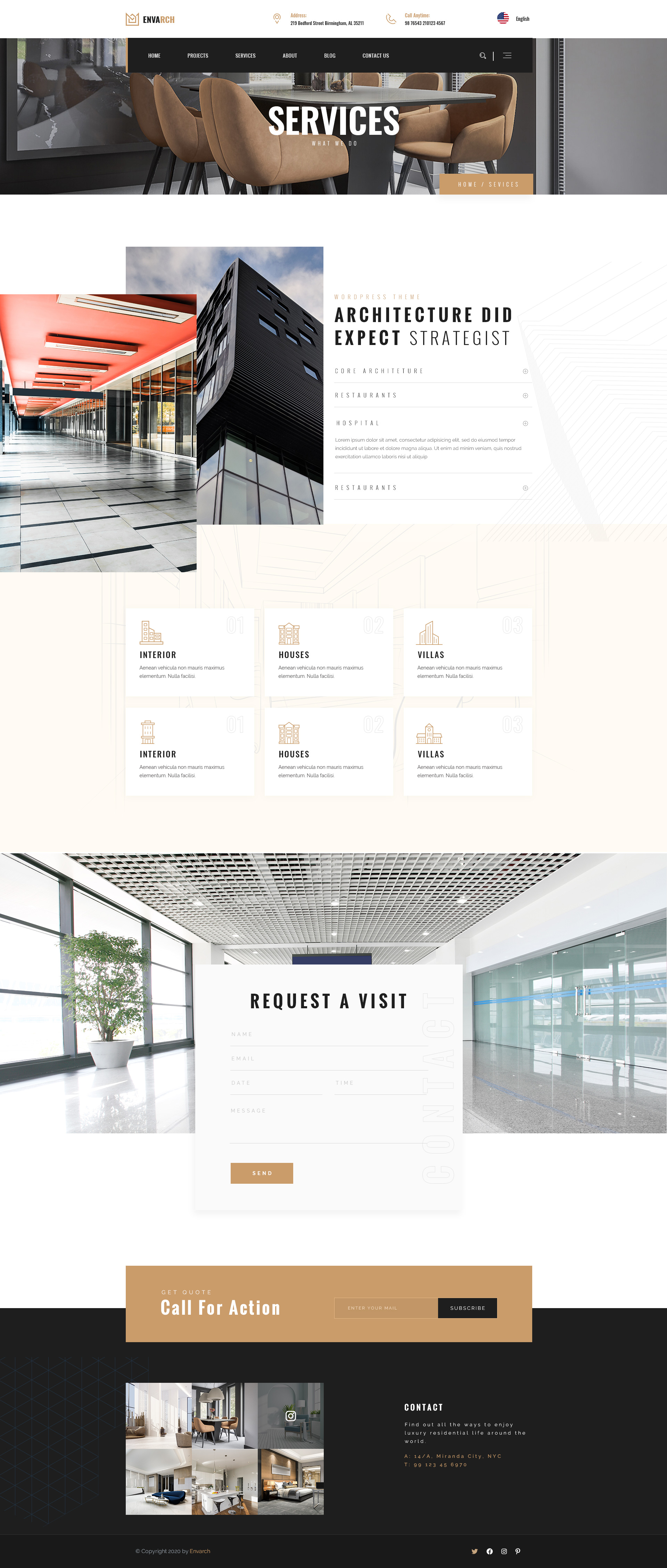Screenshot of a professional office setting featuring a neatly arranged table surrounded by brown chairs. The image prominently includes various service offerings such as architecture and strategic planning, represented by keywords like "think DIP" and "expect strategist." Six white rectangles are displayed, presumably for information input or navigation purposes. A portion of the screenshot depicts a hallway within a building with a prompt labeled "request a visit." The screenshot also features input boxes for user information alongside a yellow rectangle containing white text, which appears too small to clearly decipher. Additionally, there is an orange rectangle prominently positioned as a call-to-action button. The bottom section of the screenshot is black, with a picture displayed on the left and corresponding information situated on the right.